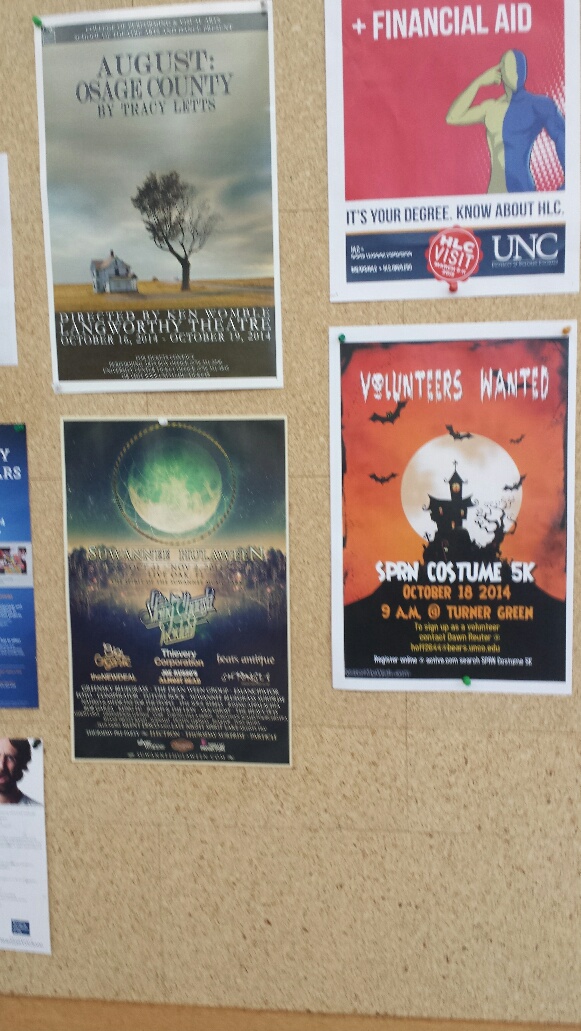This photographic image depicts a close-up view of a brown cork bulletin board adorned with four detailed posters. The top left poster promotes "August: Osage County" by Tracy Letts, directed by Ken Womble, with show dates at Langworthy Theater from October 16th to October 19th, 2014. This poster features an image of a solitary house in the countryside adjacent to a tree. Directly to the right is a vibrant red poster with the text "Financial Aid," showcasing a half-yellow, half-blue illustrated man pointing to his head. This poster also includes the phrases "It's your degree, know about HLC," an emblem stating "HLC visit," and the letters "UNC" in the bottom right corner. Beneath it, the third poster has a Halloween theme and requests "Volunteers Wanted" for a "SPRN Costume 5K" happening on October 18th, 2014, at 9 a.m. at Turner Green. This poster presents an eerie scene with a haunted house, a large moon, an orange sky, and flying bats. The bottom left poster is partially indecipherable but conveys a nighttime setting with a luminous green moon against a dark sky with trees, possibly mentioning "Hulaween." The bulletin board has additional posters on the far left edges, though they remain unreadable.